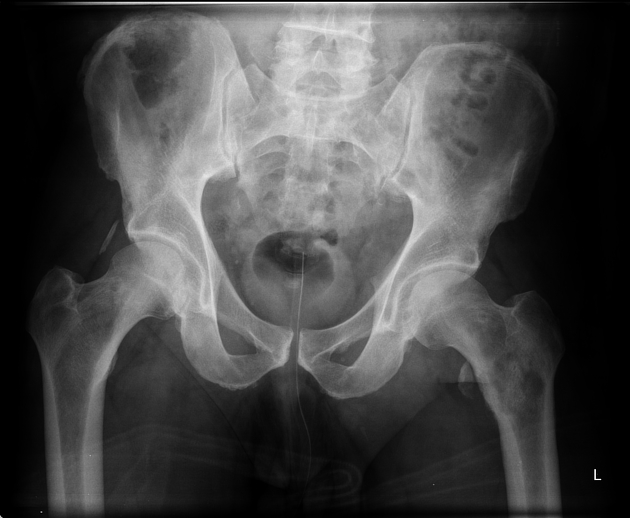This detailed X-ray image predominantly showcases the pelvis, hip bones, and surrounding structures of an individual. Prominently marked with an "L" in the lower left corner to indicate the left side, the X-ray features a stark black background, with the central focus being white, where the bones are visible. At the center, the symmetrical hip bones, pelvic bones, and part of the lower spine are distinctly highlighted. The sacrum is also visible, and surrounding parts, including the soft tissues of the muscles, appear as faded white areas. The image reveals details such as the joint areas of the hip and pelvis, making it clear that it is capturing the mid-region of a human, with no visible abnormalities noted. The hind legs are extended outwards, showing a clear, undisturbed connection with the pelvic region, and the absence of broken bones or irregularities suggests a typical X-ray of the pelvis and hips.